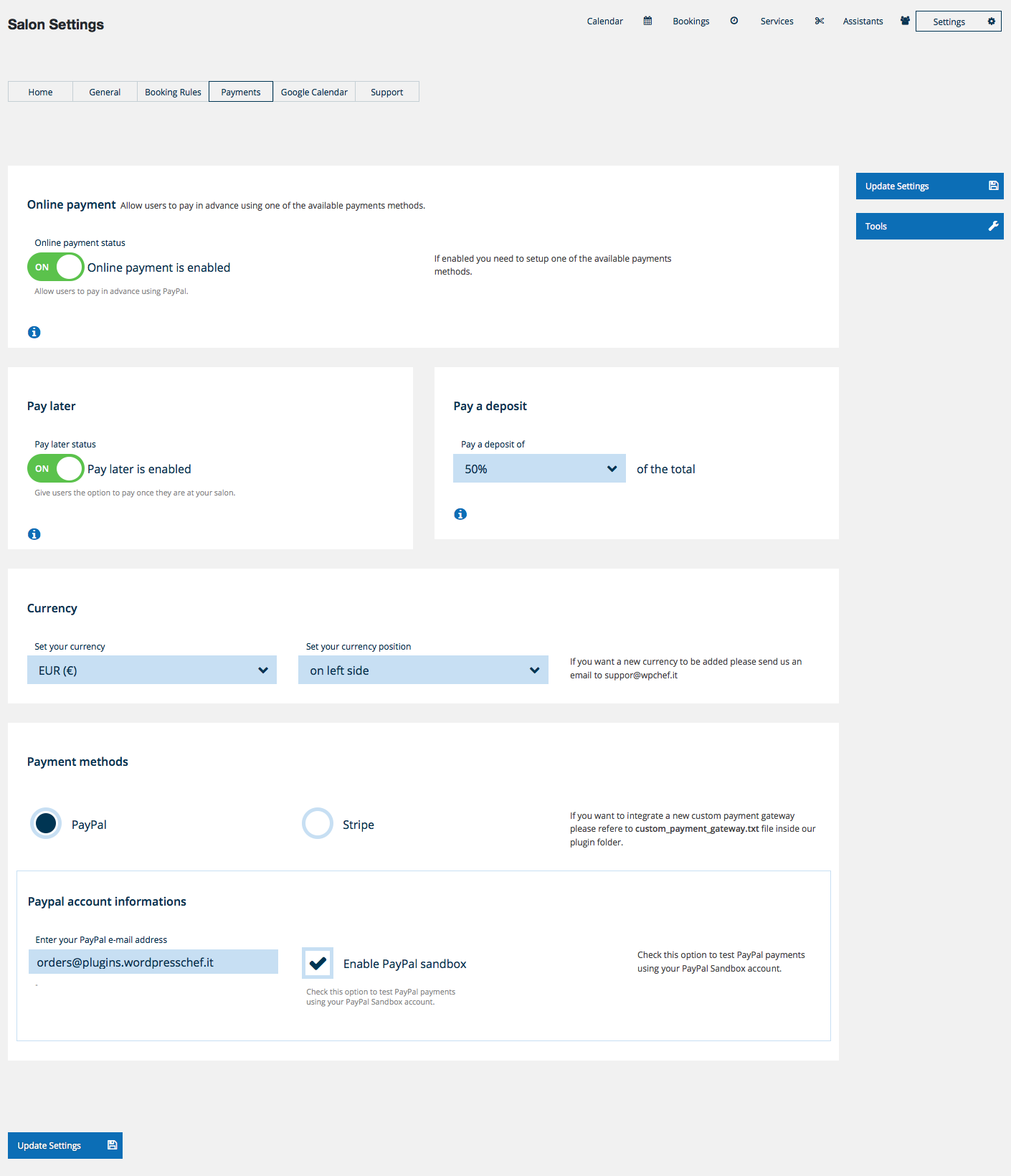A detailed screenshot of a salon management software dashboard, displayed on a desktop or laptop. At the top of the screen, the header reads "Salon Settings" in black text. To the far right, navigation options include "Calendar," "Booking," "Services," and "Assistance," indicating functionalities for managing both employee and customer appointments and services within a salon environment.

Below the header, a secondary navigation menu features tabs labeled "Home," "General," "Booking Rules," "Payments," "Google Calendar," and "Support." The "Payments" tab is currently selected.

The payments section shows various options: 
- "Online Payments" is enabled.
- "Pay Later" is also enabled.
- "Pay a Deposit" is set to 50%.
- The currency is set to Euro (€), positioned on the left side.

Under "Payment Methods," PayPal is selected, with an alternative option available via Stripe. The "PayPal Account Information" provides an email address: orders@plugins.wordpresschef.it. A checkbox labeled "Enable PayPal sandbox" is ticked, indicating that a test environment for PayPal transactions is active.